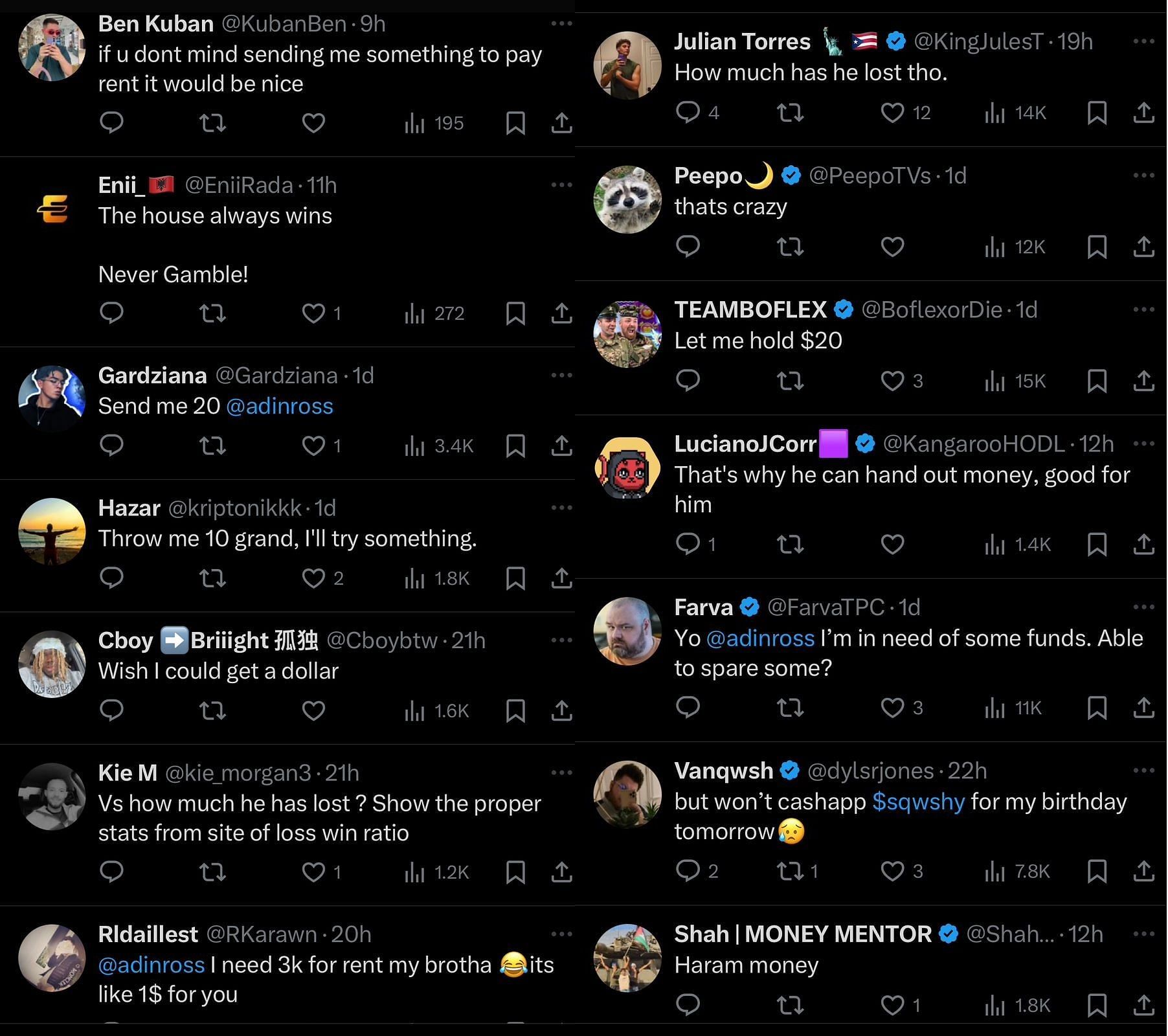This image is a square screenshot of a social media site set against a solid black background, featuring white, gray, and blue text. In the upper left corner, there is a thumbnail image of a young man wearing sunglasses, identified as Ben Kubin (@Kubin_Ben), who posted nine hours ago. His message reads: "If you don't mind sending me something to pay rent, it would be nice." Below his post is a statement from a user named Eenie that says, "The house always wins. Never gamble."

The next post is from Garziana (@Garziana), made one day ago, stating, "Send me $20 @Aiden_Ross." Beneath that, another user named Hazar (@Krypton_it) posted a day ago, writing, "Throw me ten grand. I'll try something." This is followed by a comment from a user named See Boy who posted 21 hours ago, expressing, "BTW, wish I could get a dollar."

In the bottom left corner, an individual named RLD Aillest (@KRKRON) posted twenty hours ago, addressing Aiden Ross: "I need 3k for rent my brother. It's like $1 for you."